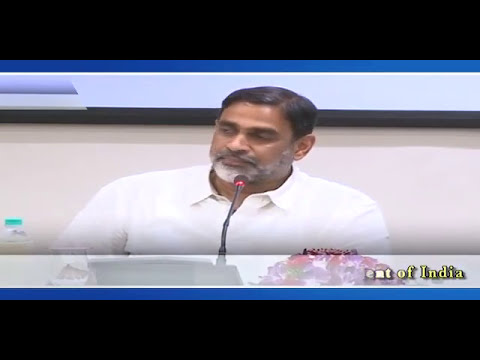This is a slightly wide rectangular screenshot from a television show, possibly a news or talk show. The image is cropped with thick black rectangular lines at the top and bottom, bordered by dark blue and grayish white transparent lines. The background is a beige wall. The man in the photo appears to be of Indian descent with dark brown hair parted on the right and a black and gray close-cropped beard and mustache. He is wearing a white or cream-colored collared shirt and is looking towards the bottom left of the camera. The man is seated and speaking into a thin black microphone, with a water bottle featuring a turquoise cap to his left and a phone in front of him. To the right of the phone is a set of flowers. In the bottom right corner, on a gray rectangle, the text "EMT of India" is displayed in yellow font. Additionally, there are strips of color across his chest, with the upper strip being white and the lower strip blue. The overall scene suggests a professional setting where the man could be discussing something significant.